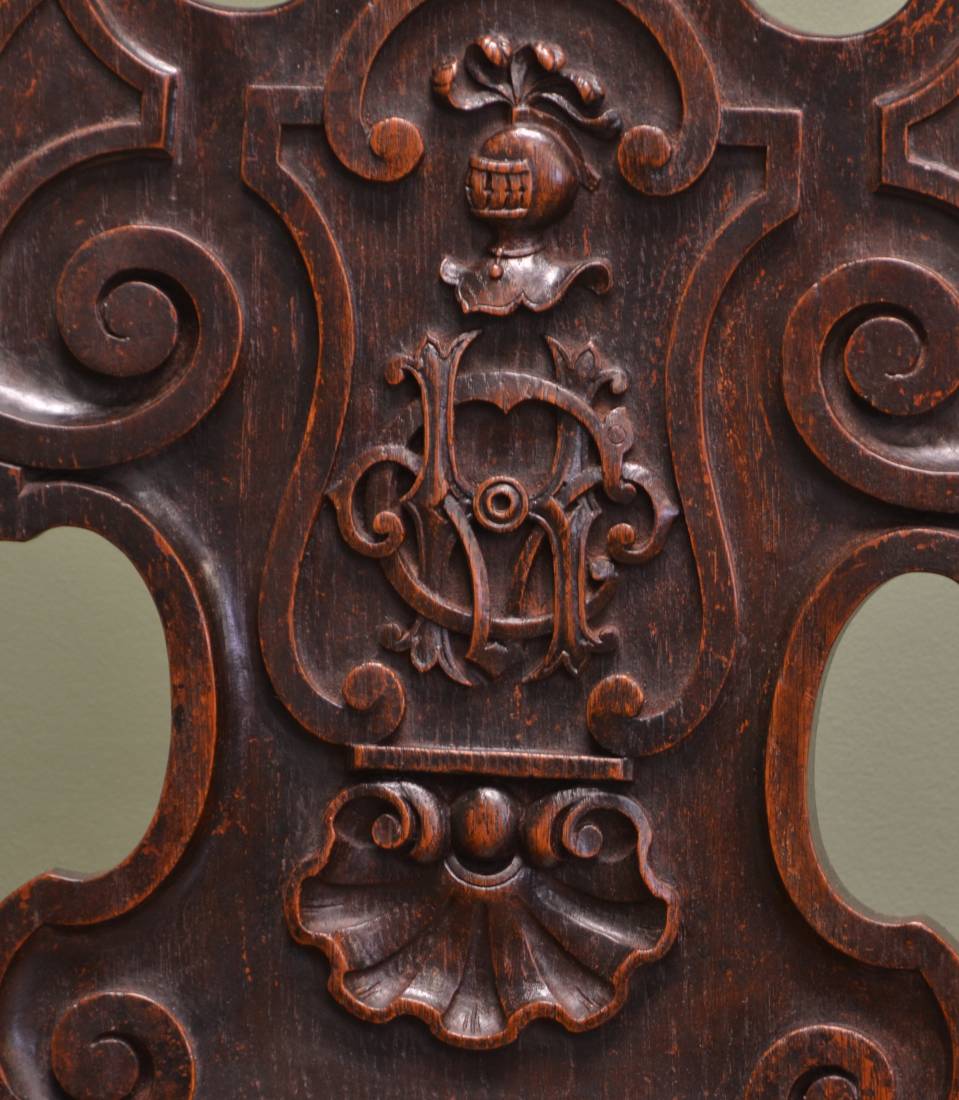This image depicts a close-up of an ornately carved, dark brown wooden object. The object, which could be part of a piece of furniture or a decorative plaque, features intricate carvings with lighter, slightly orange tones on the tips. The corners of the object are adorned with decorative swirls, creating a border around the detailed centerpiece. In the center, an intertwined monogram, possibly consisting of the letters C, H, and K, is prominently displayed. Above the monogram is the carved helmet of a knight, encased in additional swirling patterns, suggesting an older, possibly Celtic design or a family crest. Below the monogram, there's a seashell-like carving, adding to the elaborate detail. The background of the image is a sage green color, providing contrast to the rich, dark wood. The exact purpose of the object is unclear due to the zoomed-in nature of the photograph, but its craftsmanship and style indicate it is a finely detailed wooden creation.